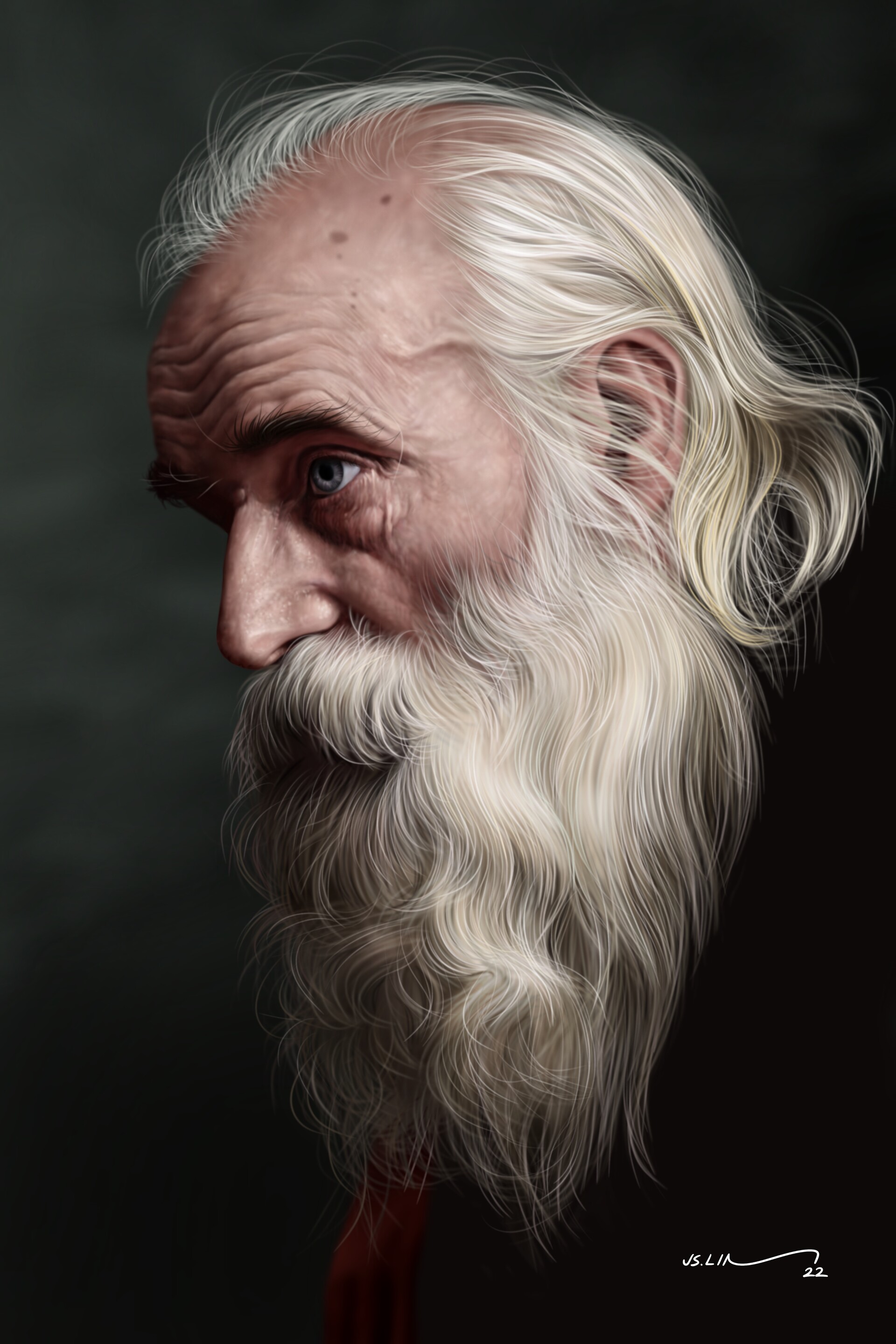This digitally-rendered portrait illustration depicts an elderly man in his 60s or 70s with a very contemplative and lost-in-thought expression. The subject is shown in profile, facing to the left, featuring his wrinkled brow and age spots. His blue-gray left eye gazes off into the distance, partially obscured by his full, flowing white beard and silky mustache. His long, white hair is slicked back but shows signs of balding on top, cascading down behind his ears and neck.

The background is a stark black and gray, creating a striking contrast against his black outfit, which blends seamlessly into the darkness. A hint of a red tie is faintly visible under his beard, adding a subtle touch of color. The image features a white signature in the bottom right corner that reads "JS Lin," followed by the number “22.” The detailed rendering makes it unclear whether it is an enhanced photograph or a pure digital artwork. The portrait orientation allows the man's head and beard to dominate the frame, emphasizing his dignified and reflective presence.